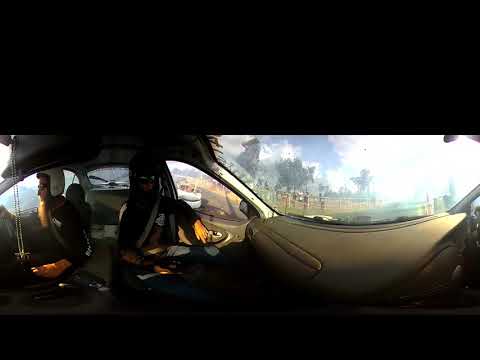The image showcases two passengers inside what seems to be a vehicle, likely elevated in the sky, possibly a helicopter. The top portion of the picture is largely blacked out, creating a significant frame that obscures a third of the image from left to right. Below this frame, the photograph appears to be a composite, merging two separate shots from within the vehicle.

On the left side of the image, occupying the leftmost 25%, a man faces left, seated and wearing a white helmet and glasses or sunglasses. He has a long brown beard and a long-sleeved black shirt. His right hand rests beside him near what appears to be a chain hanging from the center mirror. Behind him, a different image shows another passenger, likely a woman, facing towards the camera but with her gaze directed slightly to the right. Her face is partially obscured by a cowl, revealing only her light-skinned lower face. She wears a short-sleeved black shirt and a seatbelt, with her left arm resting on the door jamb.

Looking beyond the passengers, through the curved dashboard and window, an outside environment of tall trees and a forested area is visible under a cloudy blue sky. There are touches of fencing and greenery that extend the scenic view. Overall, the composite image, framed with significant black sections, illustrates a dynamic, multi-layered scene of flight over a lush, natural landscape.